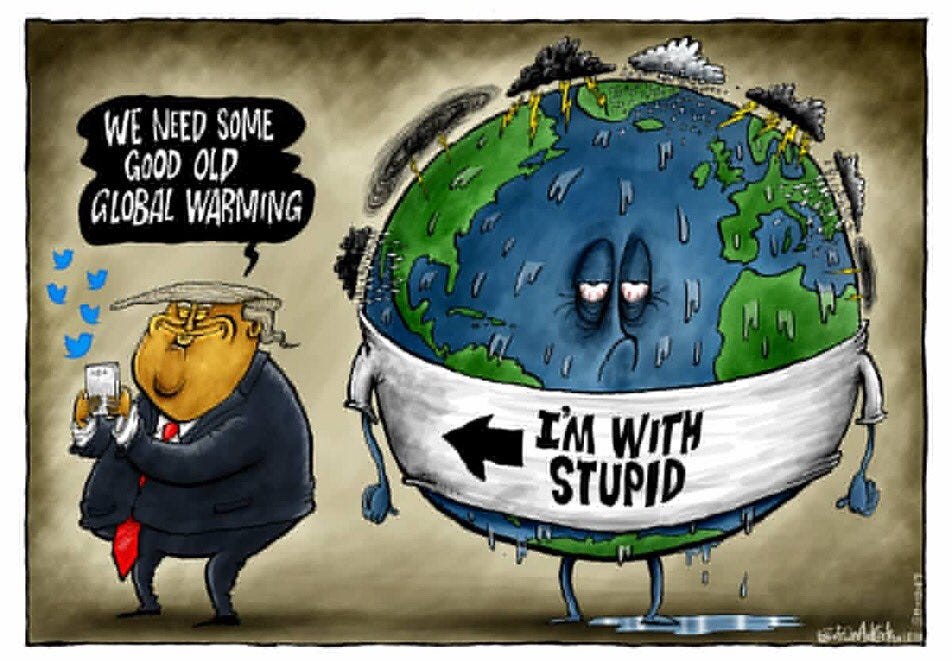This cartoon image presents a satirical scene featuring an obese caricature of Donald Trump on the left and a personified, crying globe on the right. Trump is depicted with exaggerated features, such as a large face, an enormous amount of blond hair, and a blue suit with a red tie extending almost to his knees. He is engrossed in his cell phone, from which numerous small blue Twitter birds emerge, symbolizing his frequent tweets. Above him, a black speech bubble with white text reads, "We need some good old global warming."

On the right side, the globe displays a sorrowful expression, with half-open, bloodshot eyes, a pronounced frown, and water dripping from it, as if it were sweating. Dark, stormy clouds loom overhead, punctuated by lightning bolts. A white banner on the lower part of the globe bears the statement, "I'm with stupid," with an arrow pointing towards the Trump caricature. The scene's backdrop is an aged, burnt-looking texture, featuring hues of dark green and yellow, enhancing the overall distressed appearance of the image.